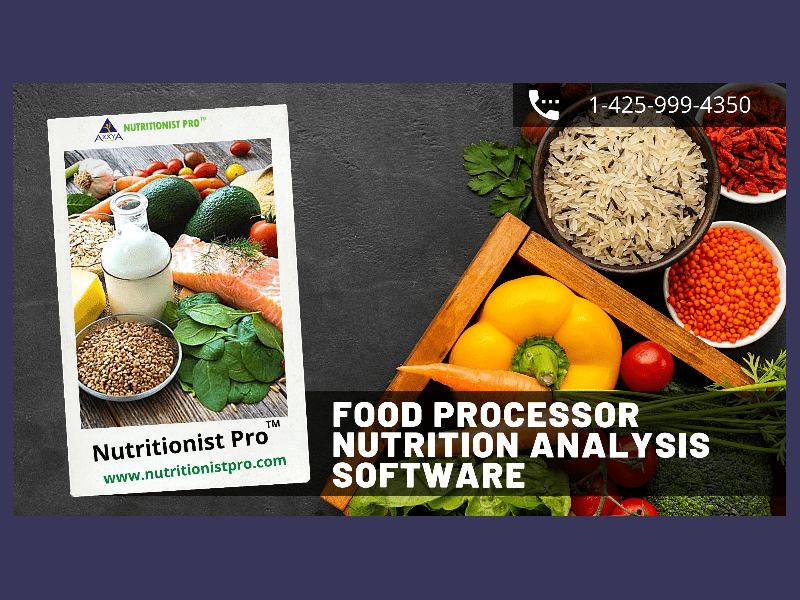The image is a detailed color photograph in landscape orientation, focusing on a variety of fresh, healthy food items displayed inside a medium brown wooden crate and on the surrounding black countertop. The crate contains vibrant vegetables including cherry tomatoes, carrots, yellow peppers, green stems, parsley, radishes, and broccoli. Adjacent to these are small bowls holding orange lentils, dried red tomatoes, red chilies, white and black wild rice grains, and possibly other grains or legumes.

To the left of the crate, there is a white publication cover tilted slightly to the left, showing an assortment of nutritious food items. This includes avocados, fresh salmon fillets, spinach leaves, cherry tomatoes, garlic cloves, a glass bottle of milk, and a clear bowl of nuts, all arranged on a wooden table. This publication cover has the title "Nutritionist Pro" written in black text, with the URL "www.nutritionistpro.com" in green beneath it.

Overlaying the image are two semi-transparent black text boxes: one at the bottom right corner that reads "Food Processor Nutrition Analysis Software" in white text, and another at the top right corner displaying the phone number "1-425-999-4350," accompanied by a small white phone icon. This intricate composition blends photographic realism with graphic design elements, emphasizing the integration of fresh food imagery with professional nutritional software branding.